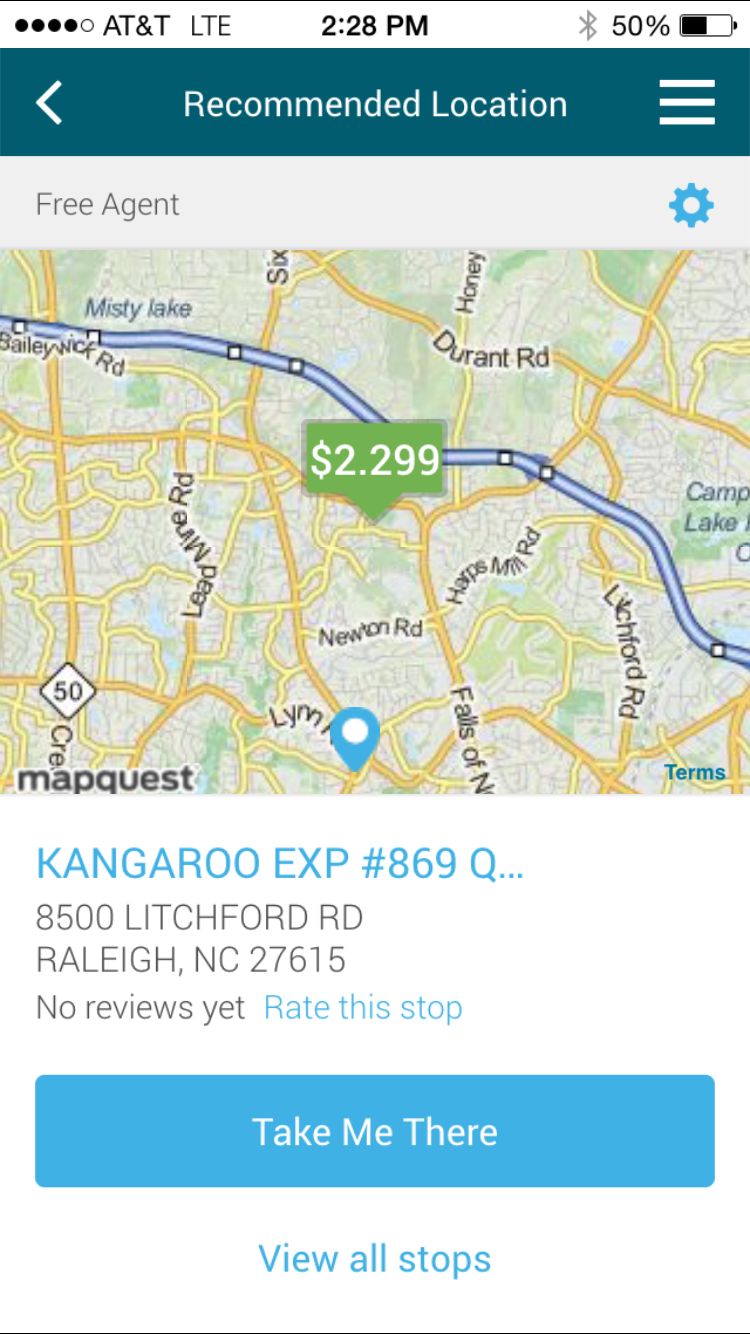The image depicts a smartphone screen displaying a recommended location. The screen is split into several distinct sections, each providing detailed information. The main focus is a map showing various geographical features such as lakes, roads, and green areas. Prominently displayed is a price tag of $2.299.

Below the map, the address of the location is listed as "85000 Litchford Road, Raleigh, NC 27615." The place is identified by what appears to be a unique identifier, "KangarooExp-869Q".

Despite being listed on the app, this location currently has no user reviews. However, there is an option to rate and review the location via a provided link. Underneath this, a conspicuous, large blue button with white capital letters reads "Take Me There," enabling users to navigate to the location. Further down, a similar-sized button with blue text on a white background reads "View All Stops."

Additionally, the top part of the screen displays various status icons, indicating the current time as 2:28 p.m., Bluetooth connectivity, and a battery level at 50%.